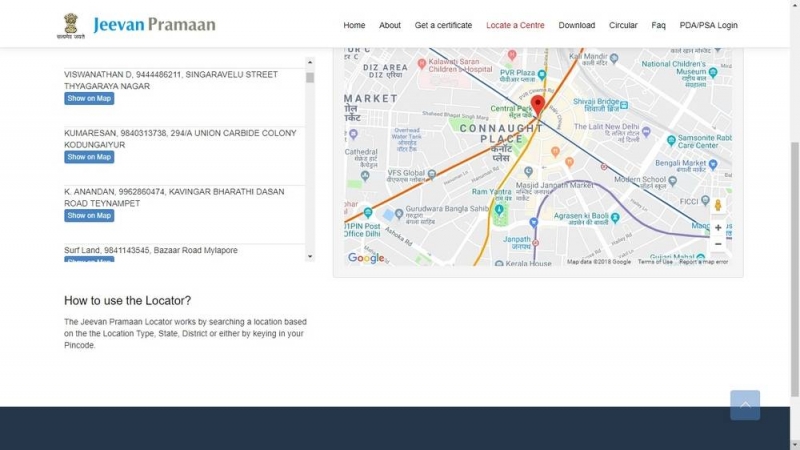This image, sourced from a website, prominently features a detailed map with a red pin marking a central location. To the left, the text "Jivin Praman" is displayed. The map highlights various significant landmarks, including a market, a cathedral, a children's hospital, Central Park, PVR Plaza, VFS Global, Jan Goff Market, Shavila Bridge, the National Children's Museum, a care center, Bengali Market, Modern School, FICCI, and several other notable locations. Additionally, there is a list of addresses on the left side of the image, each accompanied by a "Show on Map" link in blue text for easy navigation.